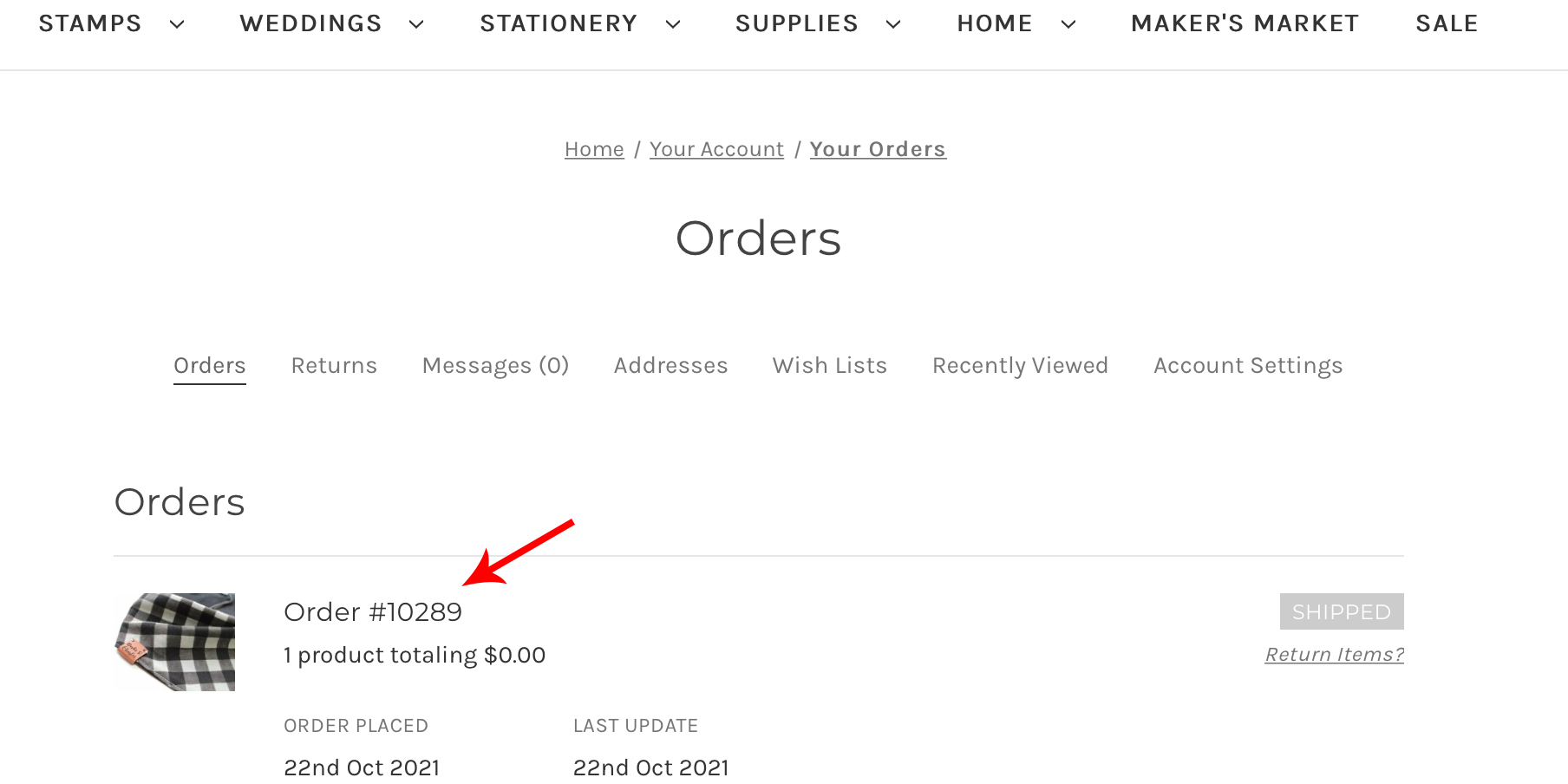Screenshot Description: The screenshot captures an orders page from an e-commerce website. At the top of the page, there's a menu bar with seven tabs: Stamps, Weddings, Stationery, Supplies, Home, Maker's Market, and Sale. Each tab except for Maker's Market and Sale has a down arrow next to it, indicating a dropdown menu.

Below the menu bar, there is a secondary navigation bar featuring three underlined options: Home, Your Account, and Orders, with the 'Orders' option in bold, indicating that the page is currently displaying order information. 

Further down, a third menu bar specifically related to order management is visible. This bar includes the options: Orders, Returns, Messages, Addresses, Wishlists, Recently Viewed, and Account Settings.

The main part of the page highlights Order #10289, which is marked by a red arrow. This order features a black and white plaid scarf, listed as one product totaling $0. The order originated on October 22, 2021, with the last update also occurring on the same date.

Next to the order details, there's a gray "Shipped" button, and to the right, an option labeled "Returned Items" is visible, indicating that the item was returned.